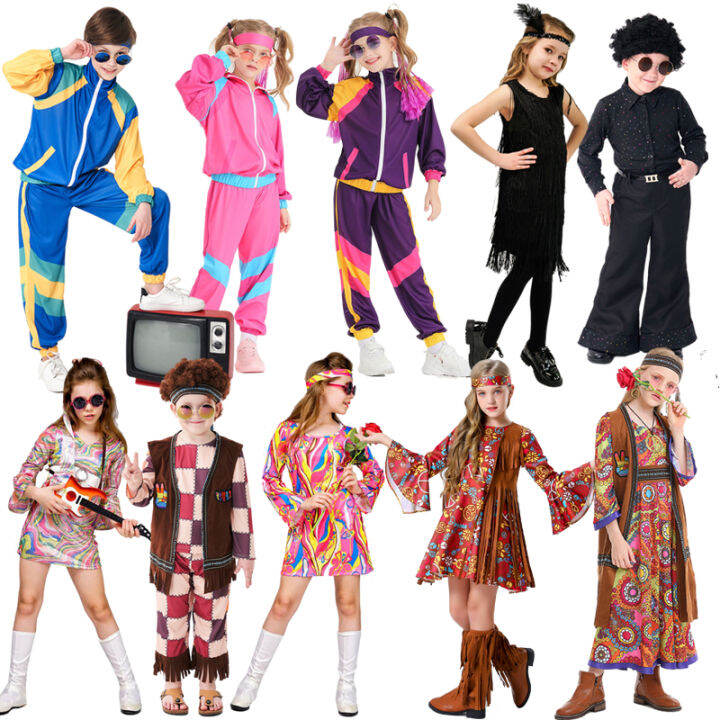The image features two rows, each containing five photographs of children dressed in costumes, likely themed for Halloween. In the top row, starting from the left, there's a boy in sunglasses and a tracksuit reminiscent of the 1980s. He is followed by two girls also in tracksuits, one of whom is wearing sunglasses. The fourth child in the row is a girl dressed in a 1920s outfit. 

The bottom row showcases kids in 1960s-style attire, embodying a hippie aesthetic. On the left, a girl is dressed in a 1960s-inspired outfit while playing a guitar. Nearby, another child is holding a flower, possibly a rose, and a boy flashes a peace sign, contributing to the flower child theme. Vibrant colors permeate the entire photo, adding to the lively, nostalgic atmosphere.